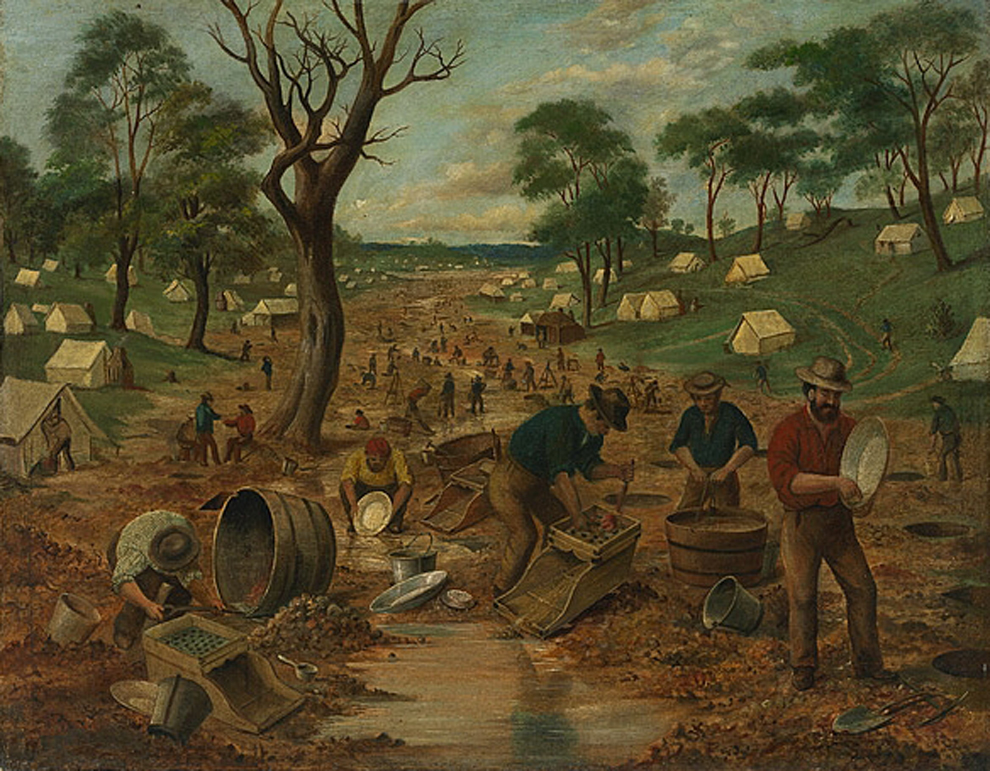This painting depicts an early 1900s scene of men working along a muddy riverbed, likely panning for gold or gems. The canvas, slightly wider than it is tall, illustrates a bustling environment with a brown trail cutting through the middle, swarming with men dressed in period-appropriate attire. They wear brown long pants, brown boots, and collared shirts in various pastel shades ranging from orange to teal. These men are engaged in various activities, using steel pans, wooden sifters, and barrels to process materials they’ve extracted from the stream bed. Although primarily men, one figure shows some feminine characteristics. On either side of the trail, white temporary huts and tents are set up within the lush, green grassy areas, which also feature sparse trees. The overall tone of the painting is quite dark and earthy, with a palette dominated by muddy browns and greens, enhancing its depiction of a rugged, labor-intensive environment.